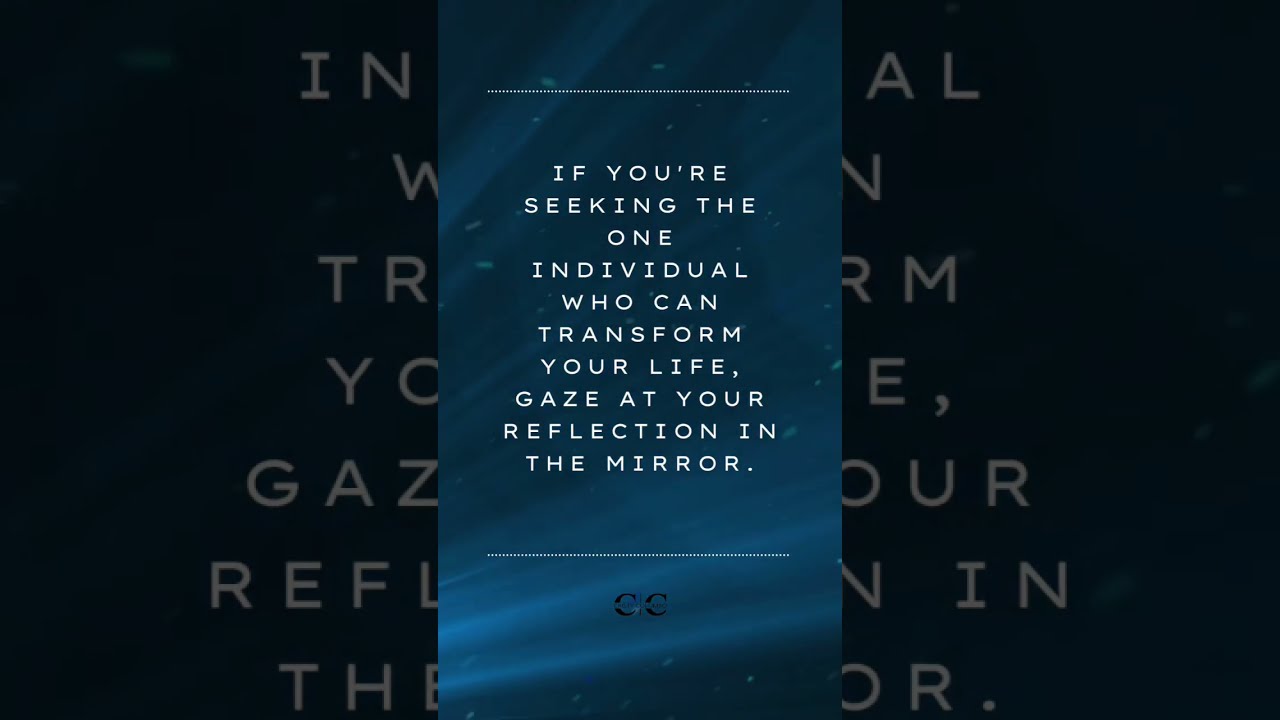The image appears to be a stylized graphic, possibly a smartphone screenshot, designed with a layered effect—a picture within a picture. The primary feature of the image is a quotation rendered in capital white letters against a dark, ocean-blue background interspersed with various shades and whitish streaks, resembling clouds or jet streams. Tiny white dots align horizontally at both the top and bottom, framing the quote which reads: "If you're seeking the one individual who can transform your life, gaze at your reflection in the mirror." Below the bottom dotted line, a watermark of two black capital C's is present. The overall composition suggests this could be a slide from a digital presentation or an Instagram story, emphasizing the message of self-empowerment.